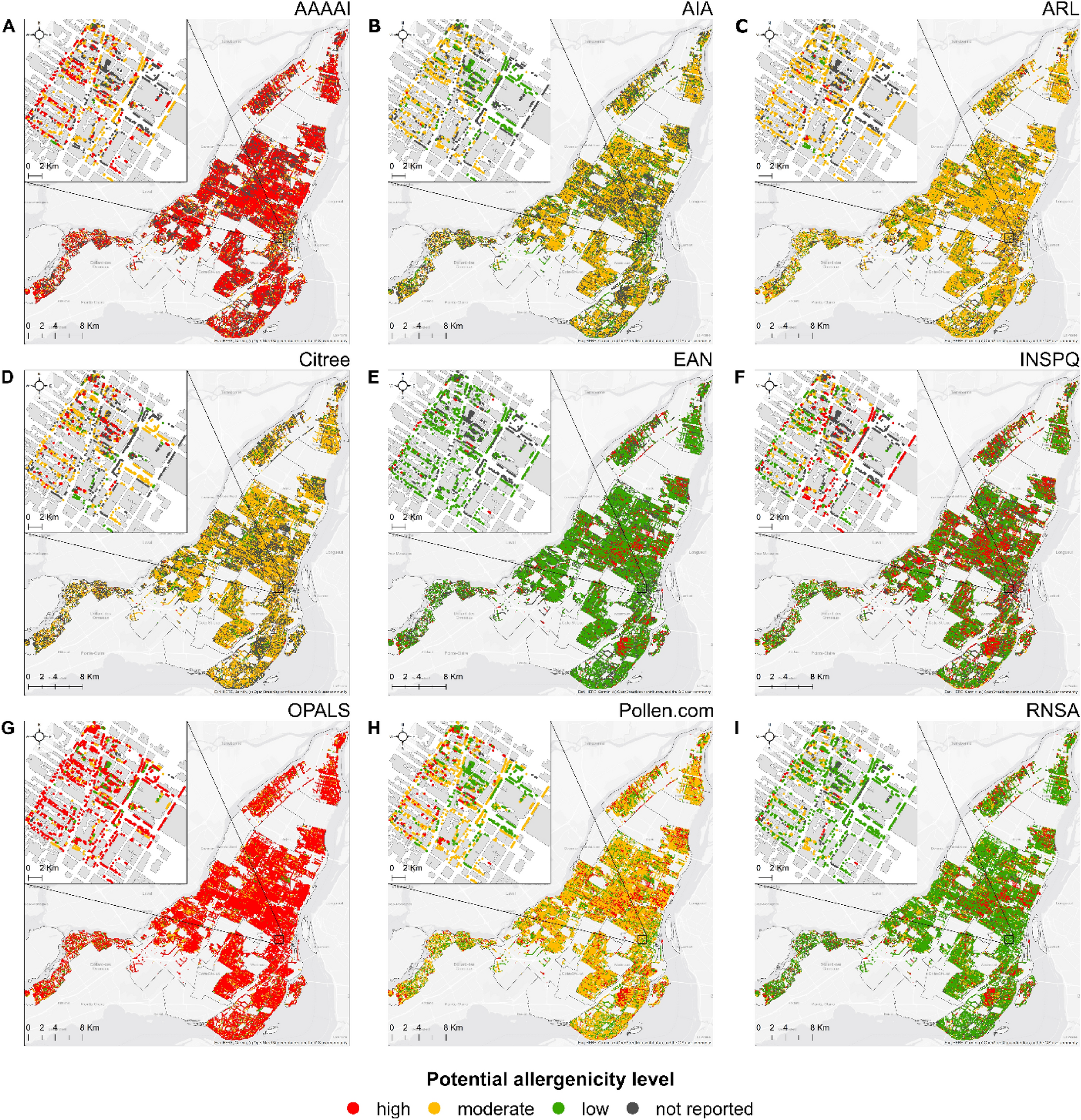This image is a detailed map comprised of nine square quadrants arranged in a 3x3 grid, each quadrant representing a different potential allergenicity level. At the bottom, a legend explains the color code: red indicates high allergen levels, yellow indicates moderate levels, green indicates low levels, and gray indicates areas not reported. The quadrants are labeled with coordinates ranging from A to C horizontally and A to G vertically, with each map displaying various colors to represent allergenicity.

In the first row, from left to right: 
- Quadrant A is predominantly red.
- Quadrant B has a primarily gray background with a lot of yellow and some green.
- Quadrant C has a gray background and is mainly yellow.

In the second row:
- Quadrant D is primarily yellow with some green.
- Quadrant E is mostly green with some red patches.
- Quadrant F is roughly half green and half red.

In the third row:
- Quadrant G is mainly red with a bit of yellow.
- Quadrant H is primarily yellow with some red and green spots.
- Quadrant I is chiefly green with some scattered red.

Each map seems to resemble the shape of a lobster and contains various letters that may indicate specific allergens or locations, such as "A" in the upper left corner, "E, A, N" to the middle right, and "I, N, S, P, Q" at the bottom. The first column of maps follows a red-yellow-red pattern, while the second column displays yellow-green-yellow with some red, and the third column shows yellow, then a mix of green and red, and finally mostly green. The detailed letters and labeled squares suggest these maps are measuring allergen levels across different regions.